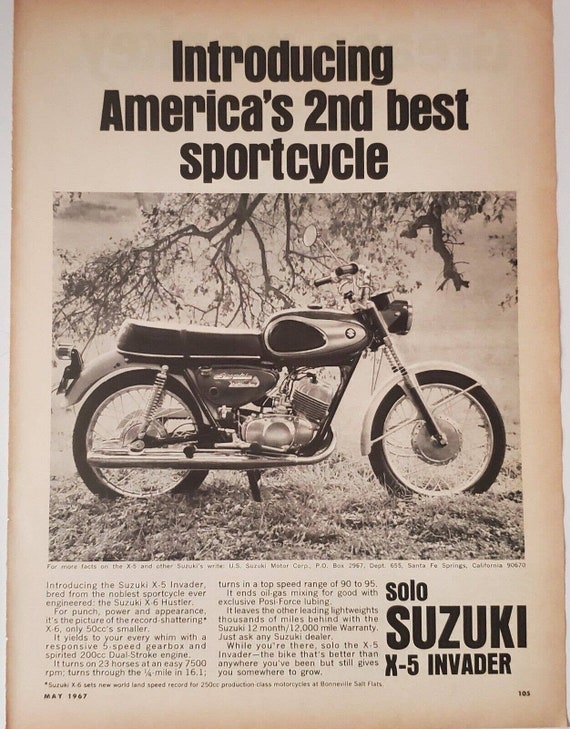The image presents a scanned, slightly aged page from a May 1967 magazine, specifically page 105, as indicated in bold black text in the bottom left and right corners respectively. The top center of the page features the headline "Introducing America's Second Best Sports Cycle" in stacked black text over three lines. Below this headline, there is a large, clear black and white photograph of the Solo Suzuki X5 Invader motorcycle, positioned in a grassy field under a low-hanging tree branch. The motorcycle's profile is fully visible, showcasing its flat seat, short handlebars, and wheel protectors. The background is a natural setting with numerous trees, emphasizing the motorcycle's presence and design. To the left of the image, there's textual content arranged in two columns detailing the model, highlighting its lineage from the Suzuki X6, and its features such as the top speed range of 90 to 95 mph and its efficient posi force lubing system that dispenses with the need for oil-gas mixing.